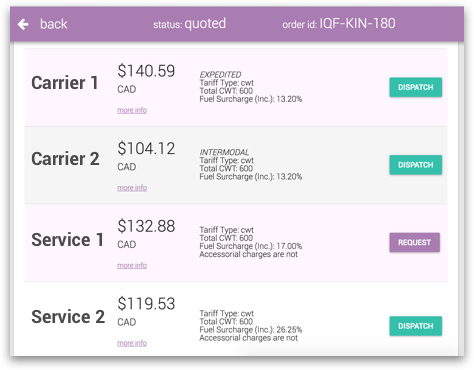This is a detailed screenshot of a mobile carrier order screen. At the top of the screen is a prominent purple banner. On the left side of the banner is a left-pointing arrow paired with the word "back" in lowercase letters, both in white. Centrally located within the banner is a status label in small white text followed by a quote in larger white lowercase letters. To the right side of the banner, the text "Order ID" is displayed, along with the specific order ID number.

Immediately below the purple banner, the background transitions to white. The top line features "Carrier One" in large black letters accompanied by the carrier's number. To the right of this text, the price is displayed. Below the price, the phrase "More Info" appears in purple letters. To the right of this section, additional service details are provided, including "Expedited Tariff Type" and "Total Fuel Surcharge." On the far right side, a bright green button labeled "Dispatch" is prominently displayed.

The section below follows a similar structure, listing "Carrier Two," along with services under it indicated as "Service One" and "Service Two." Each service is formatted with the price listed first, followed by the product description. For "Service One," there is a button labeled "Request." For "Service Two," similar to the earlier section, a "Dispatch" button is also provided.